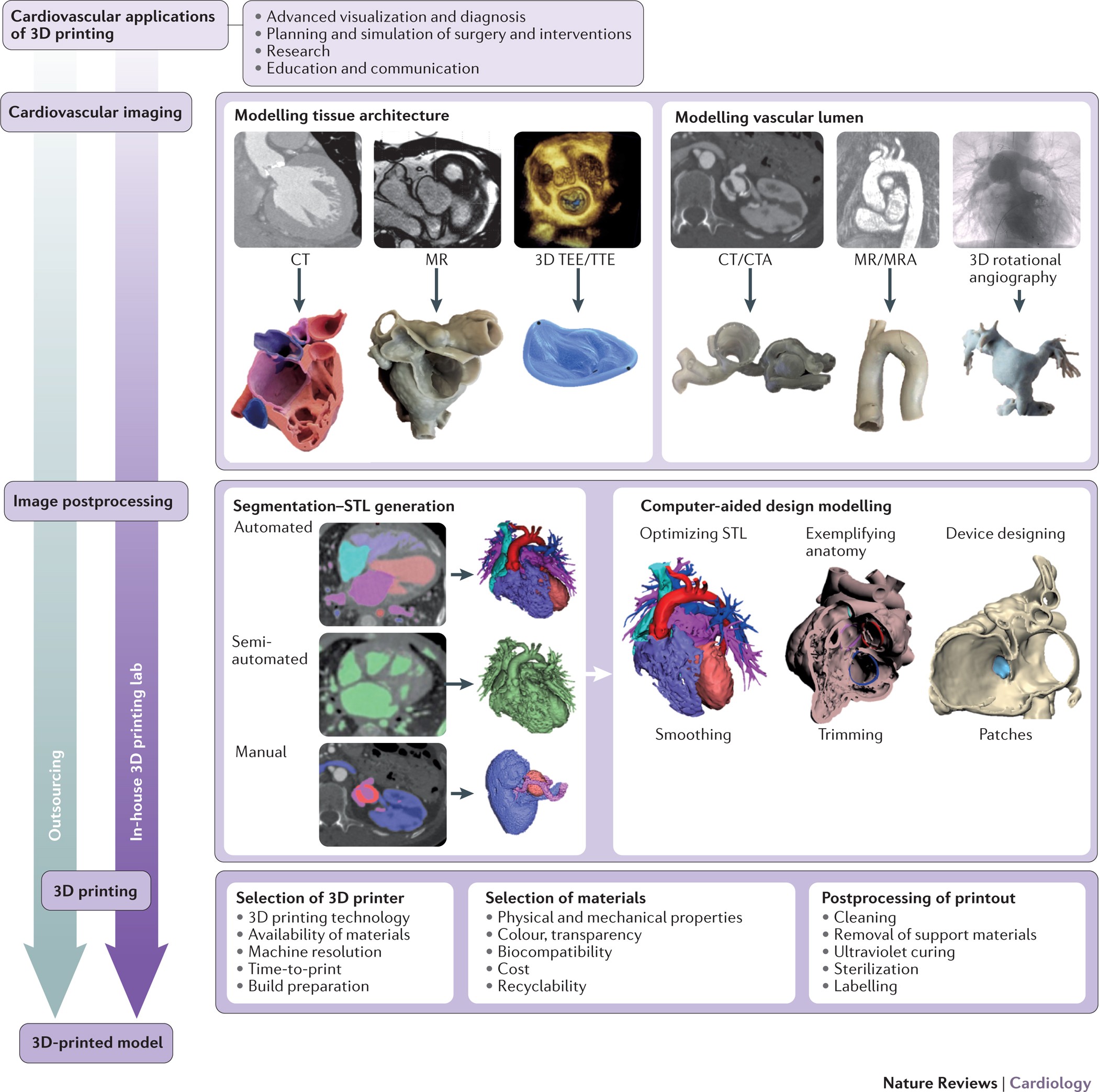The image is a detailed educational infographic from the scientific journal Nature Reviews Cardiology, likely appearing in a medical textbook. It showcases the cardiovascular applications of 3D printing through a montage of both photographic and illustrated images. At the top, lavender text boxes highlight key uses: Advanced Visualization and Diagnosis, Planning and Simulation of Surgery and Interventions, Research, Education, and Communication.

Several rows of white boxes exhibit the step-by-step process, starting with cardiovascular imaging, including cross-sectional views and 3D visualizations of the human heart and vascular structures. Labels such as Modeling Tissue Architecture and Modeling Vascular Lumen accompany these images. Under the heading Image Post Processing, concepts like Segmentation, STL Generation (Automated, Semi-Automated, and Manual) are illustrated, along with subsequent visualizations of the heart.

The infographic follows a flowchart that maps out the journey from initial imaging to the final 3D printed models. This includes Computer-Aided Design (CAD) Modelling for optimizing STL files, exemplifying anatomy, and designing devices like arterial patches. The selection of the 3D printer is discussed in detail, covering 3D printing technology, machine resolution, the time requirement to print, availability of materials, and build preparation.

Further, the selection of materials is broken down into physical and mechanical properties, color, transparency, biocompatibility, cost, and recyclability. The final section, Post-Processing of Printout, outlines steps such as cleaning, removing support materials, ultraviolet curing, sterilization, and labeling. The comprehensive presentation uses variously colored hearts and clearly delineated arrows to depict the transformation from medical images to detailed 3D printed models, emphasizing the innovative utility of 3D printing in cardiovascular applications.